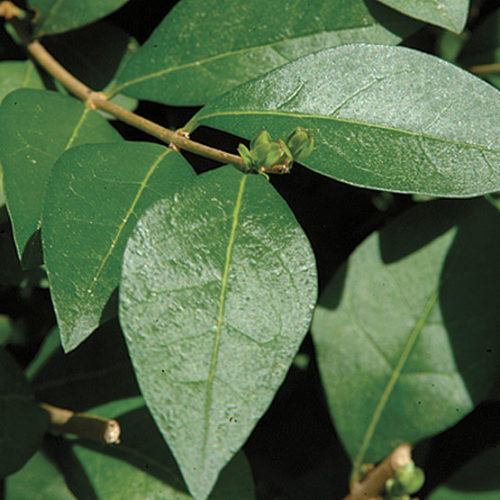This vibrant and detailed nature photograph captures a close-up of a plant stem, showcasing the intricate beauty of its green, teardrop-shaped leaves on a sunny day. The setting is outdoors, bathed in the natural sunlight that cast glossy reflections on the lush foliage, suggesting it was taken in late spring or early summer. The main stem, which has a light greenish-brown hue, prominently features a cluster of five to six simple, tapered leaves radiating from the center. At the tip of the stem in the middle of the image, there's a subtle but notable green bud that blends into its surroundings, hinting at potential new growth or perhaps a small, camouflaged green frog perched delicately at the end. The edges of the photo also reveal some out-of-focus elements: in the lower right corner, an indistinct stem, and in the lower left corner, a cut or snapped branch with visible pulp, adding depth and texture to the scene.